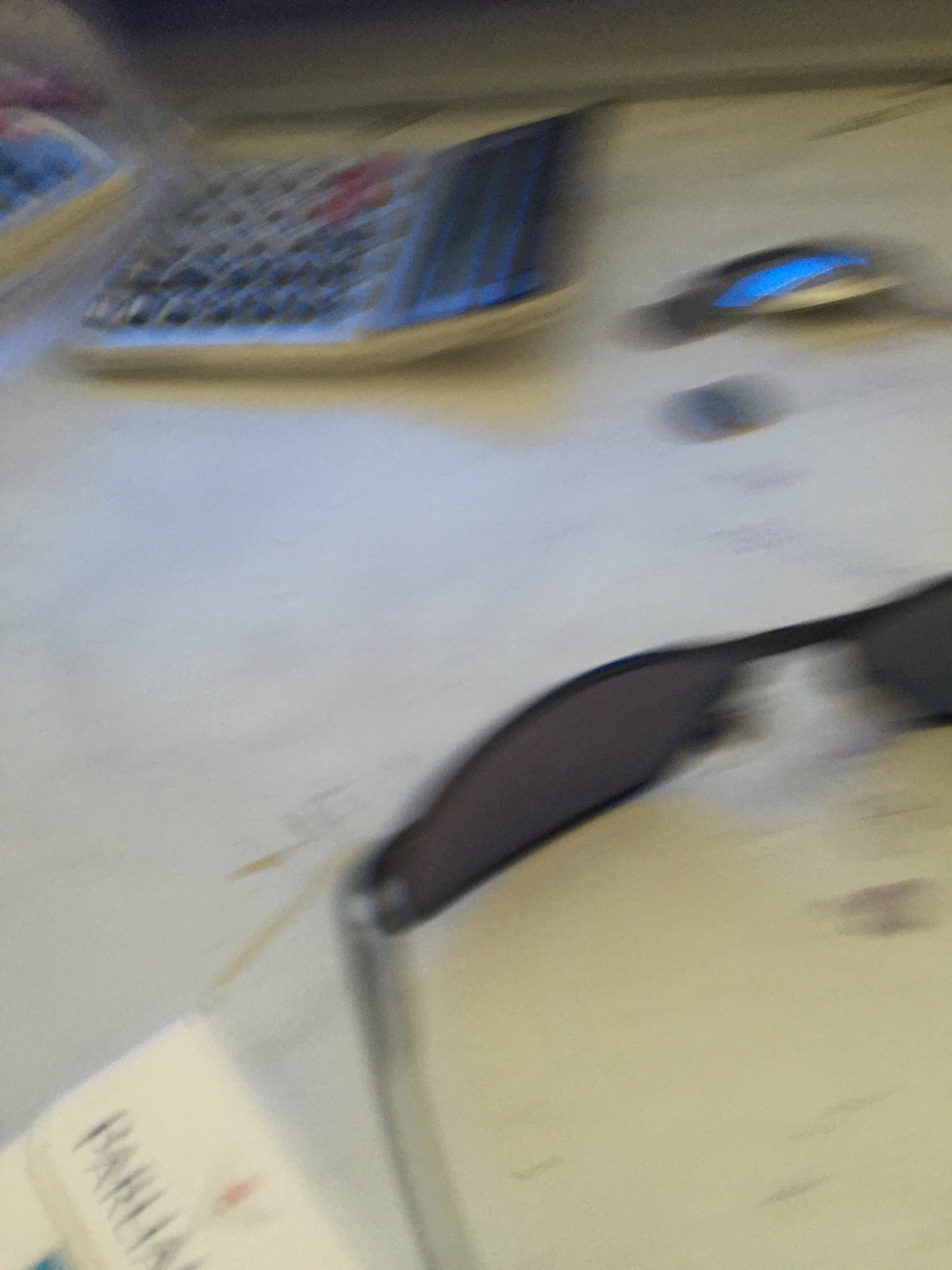In this image, a heavily blurred photograph depicts what seems to be a countertop or tabletop, possibly composed of white material with indistinct gray veining reminiscent of marble. Despite the blur, several objects are discernible on the surface. Positioned towards the top left, a silver-colored calculator is visible, marked by a mix of dark and light-colored buttons, although the specifics are obscured by the blur. Near the bottom-center of the image, a pair of sunglasses with dark lenses can be identified, with the arms appearing to be of a lighter hue. The image is devoid of any textual elements.